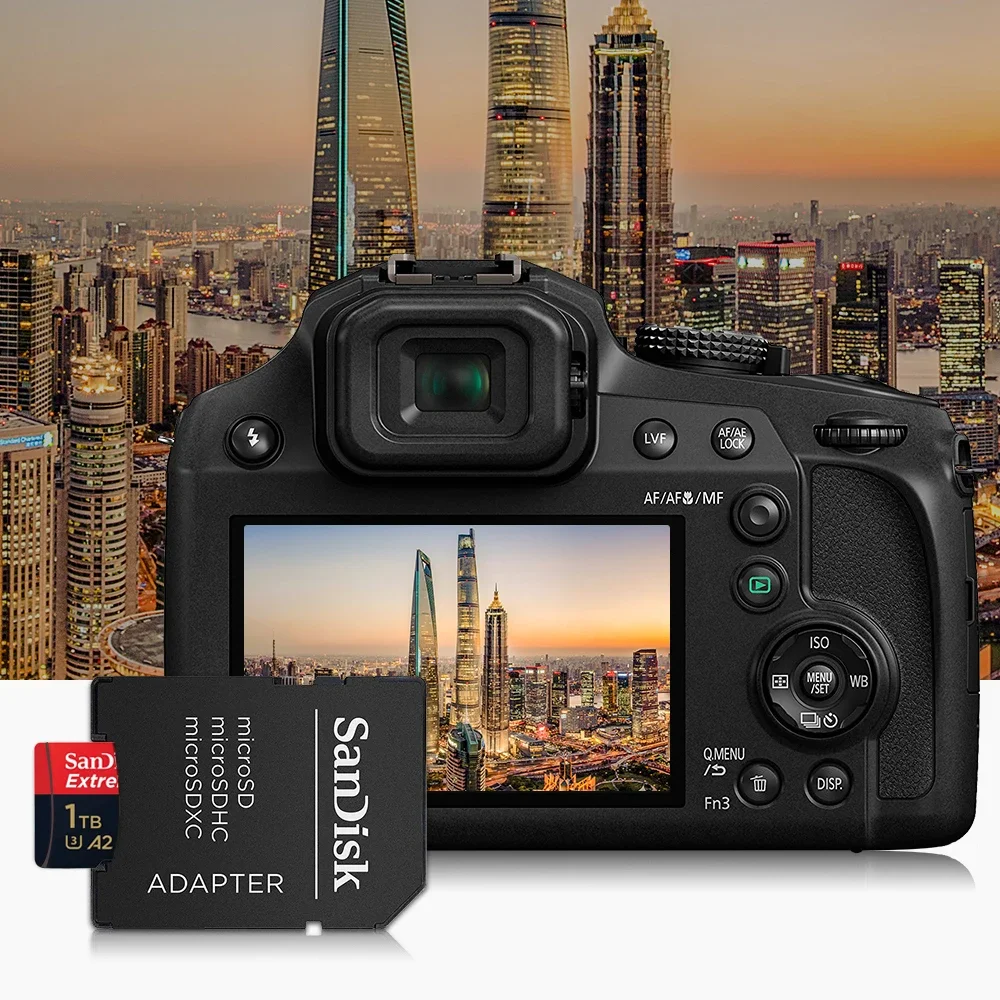The photograph showcases a meticulously detailed advertisement featuring SanDisk microSD cards and adapter. Dominating the foreground is a sleek black digital SLR camera, with a crisp and clear display screen. Prominent on the screen is the image of a vibrant cityscape, captured at sunset, with illuminated skyscrapers and a river visible in the background. The tallest building on the left side of the skyline is distinctly marked by a blue line running vertically. Obscuring part of this scenic view is an SD card adapter from SanDisk, prominently placed over the bottom left of the camera. The adapter, lying on its side, bears the white SanDisk logo and labels for microSD, microSDHC, and SDXC. Inserted into this adapter is a black and red memory card, further emphasizing the focus on SanDisk's storage solutions. Overall, this composition highlights the synergy between advanced photography equipment and reliable data storage, set against the backdrop of a stunning urban panorama.